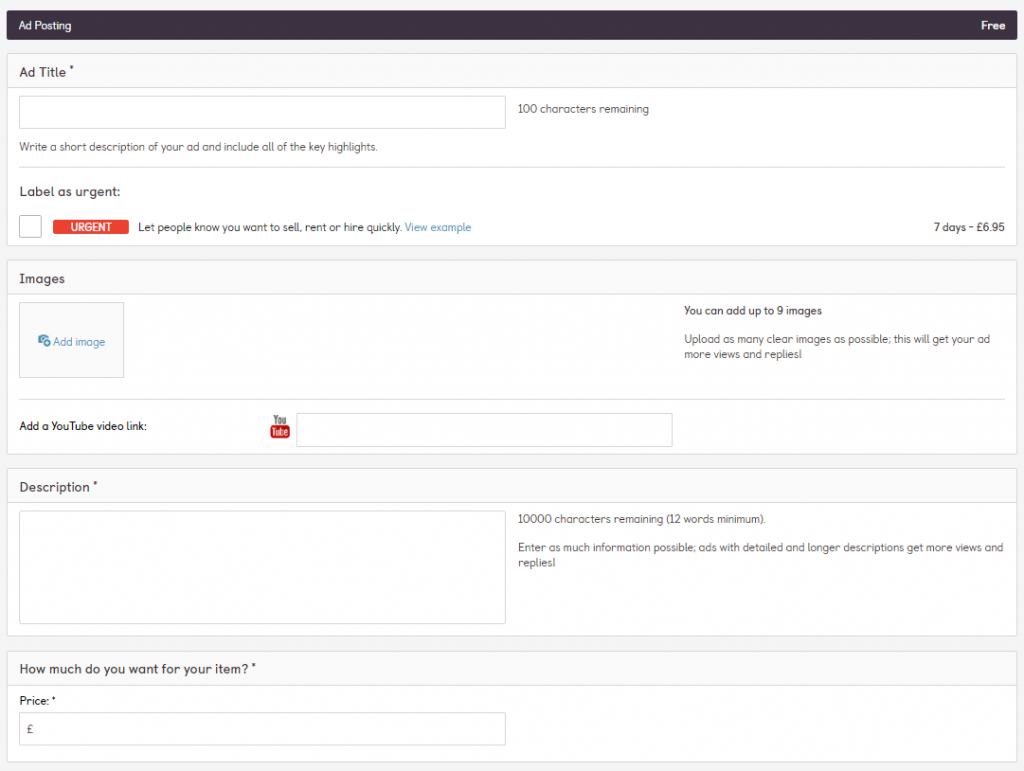This image is a highly detailed screenshot of a webpage, featuring several distinct sections and elements. 

At the very top of the image, there is a dark gray rectangular header with slightly rounded corners, set against a light gray background. On the left side of this header, the white text reads "Add Posting," while on the far right side, it says "Free" in white text.

Beneath this main header and a small area of negative space, there is a pane with a white background and a light gray rectangular header. The header on the left reads "Add Title*" in dark gray text. 

Directly below the header, within the white background of the pane, is a text box positioned in the upper left corner. This text box is white with a thin light gray outline. To the right of the text box, light gray text states "100 Characters Remaining." Below this, in a similar font style, instructions are given: "Write a short description of your ad and include all of the key highlights."

Below this segment, a thin light gray line runs horizontally almost across the entire width of the pane. Underneath the line, on the left side, "Label as Urgent" is written in dark gray text. At the bottom left corner of the pane, there is a white checkbox outlined with a thin light gray line. To its right, there is a bright red rectangular button with "URGENT" displayed in all caps white text. 

Further to the right, light gray text explains, "Let People Know You Want to Sell, Rent, or Hire Quickly." Still further to the right, blue text reads "View Example."

In the bottom right corner, there is additional light gray text indicating "7 Days - £6.95."

Following another area of negative space below this pane, there is a similarly laid-out pane. Its header features dark gray text on the left side, reading "Images."

This detailed description captures the structural and textual elements of the webpage, offering a clear visual representation through words.